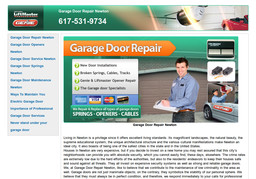A small, blurry image depicts a desktop screenshot of a garage door repair website. The image is too wide to be from a mobile device, and much of the text is indiscernible. The phone number visible on the website is 617-531-9734, and the site features two logos on the left side. Moving to the right, there is an image of a car in a garage. The website offers various garage door services including the repair of springs, openers, and cables, with a thorough check of all work completed.

The site also displays a photograph of a technician wearing a long-sleeve pullover and holding a clipboard, standing outside a garage door. Another individual is seen near a car, inspecting another garage door. The acceptable payment methods listed include American Express, Visa, MasterCard, and Discover. Navigation options on the left side of the website include links to garage door repair, garage door openers, and garage door springs, although specific text is mostly unreadable. This image captures the main elements of a garage door repair service's website.